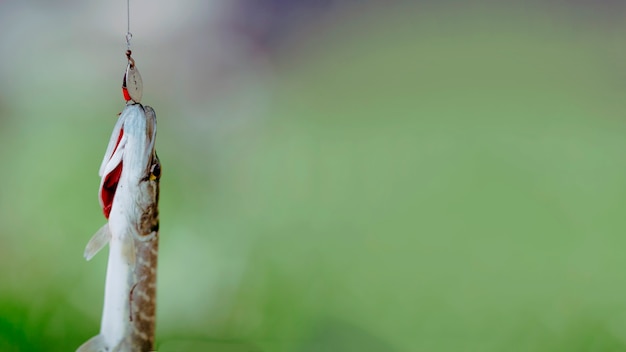In this full color, horizontally rectangular outdoor photograph, the background features a charming bokeh effect with dominant hues of green, interspersed with patches of white and hints of purple. At the lower left corner, the main focus is a small, slender fish suspended vertically from a fishing lure. The fish, with its white underbelly and golden eye, showcases distinct brown and white stripes along its top and reveals a glimpse of the red interior of one of its gills. The silver and red lure, attached to a fishing line, holds the fish in place, casting a stark contrast against the blurred backdrop. About two-thirds of the fish’s body is visible, emphasizing its delicate form against the indistinct scenery.